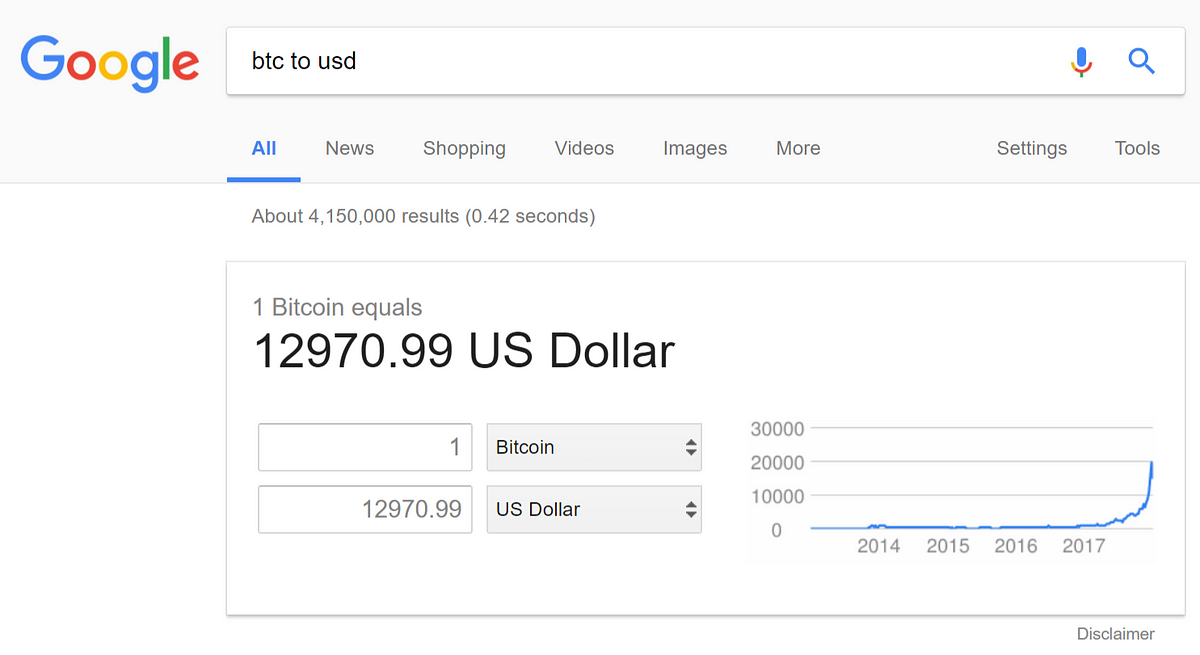In this screenshot of a Google search result, the familiar Google banner is displayed prominently at the top, featuring the iconic Google logo in a combination of blue, red, yellow, and green colors to the left. The search bar prominently reads "BTC2USD" and includes the Google microphone button, colored in blue, red, green, and yellow, next to the blue magnifying glass icon indicating search function.

Below the search bar, various tabs are visible, including "All," which is highlighted in blue with a blue underline indicating it's the current selection, "News," "Shopping," "Videos," "Images," and "More." To the right, "Settings" and "Tools" options are displayed. The search has yielded approximately 4,150,000 results in about 0.42 seconds.

A highlighted information box below the search bar indicates that "1 BTC equals $12,970.99," accompanied by a blue graph illustrating an upward trend in the cryptocurrency's value.